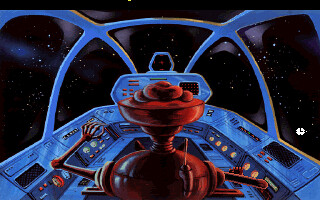The image is a detailed, artistic depiction of a science fiction scene from a computer game. It portrays the interior of a spaceship, with a rounded, crimson-metallic red robot seated in the cockpit. The robot, which possesses a rounded body, thin arms and fingers, and a head that flattens at the top with some type of items on it, is depicted from behind. The spaceship's interior is predominantly a bright metallic blue, including blue curved portions framing the windows. Various control panels filled with buttons, screens, and intricate details are visible on both sides of the cockpit. Through the spaceship's windows, the vast, dark expanse of outer space is visible, speckled with white dots representing distant stars. Additionally, there are hints of purple and blue nebulae in the backdrop, enhancing the cosmic setting. The overall scene combines both vibrant interior colors and the enigmatic beauty of space outside.